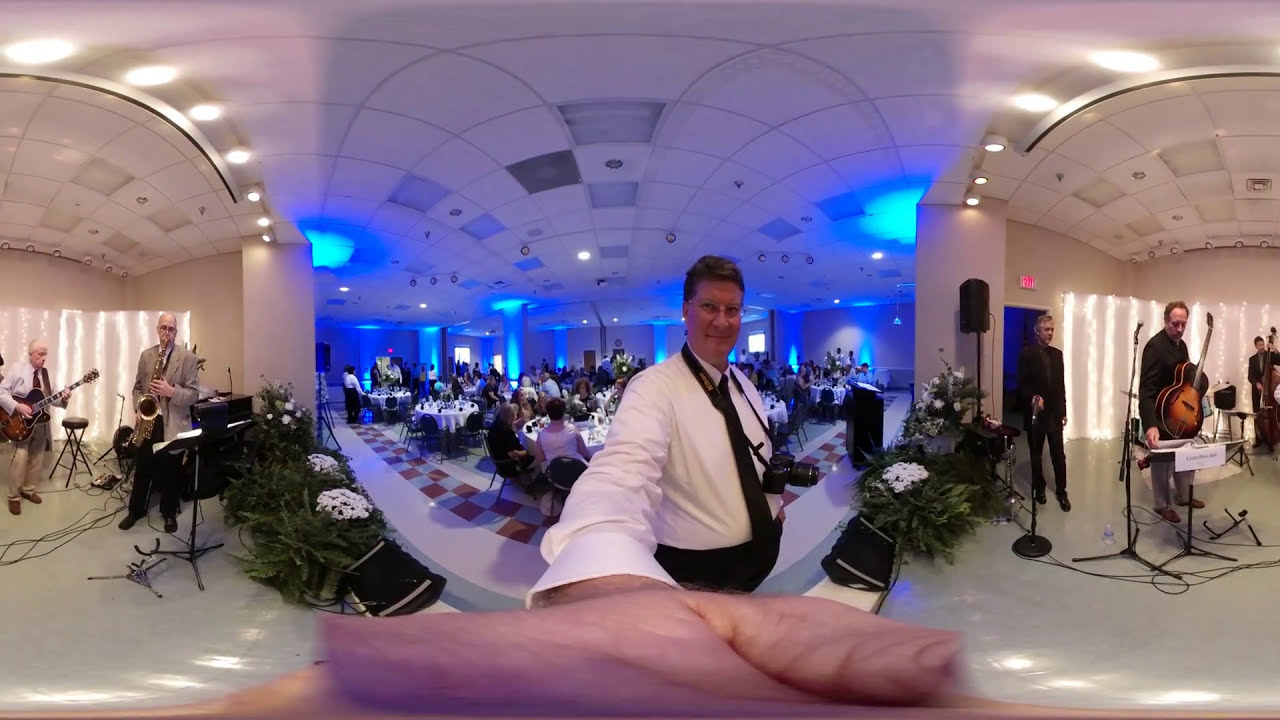In this panoramic photograph, a middle-aged man is seen taking a selfie with his right hand outstretched, holding the camera. He is dressed in black dress pants, a white long sleeve button-up shirt, and a black tie. The man is also wearing glasses and has a black camera strap around his neck, attached to a black camera with a large telephoto lens. The image, split by the nature of the panoramic shot, shows the man centered between what appears to be the same stage duplicated on both the left and right sides. 

On the raised, carpeted gray platform, multiple musicians are performing. To the left, a saxophonist and a guitarist are situated in an arched area. To the right, an electric guitarist stands behind a microphone connected with various black wires, with a brown and black acoustic guitar in hand and a music stand in front of them. Additionally, there's a bassist and a violin player further to the right. 

Behind the man, a dining hall is visible with white tablecloth-covered round tables, suggesting a formal event, possibly a wedding or special dinner, with numerous guests seated and enjoying the music. The panoramic effect makes the stage appear split across two rooms, but it likely encompasses a single space viewed from the guests' perspective facing the musicians.